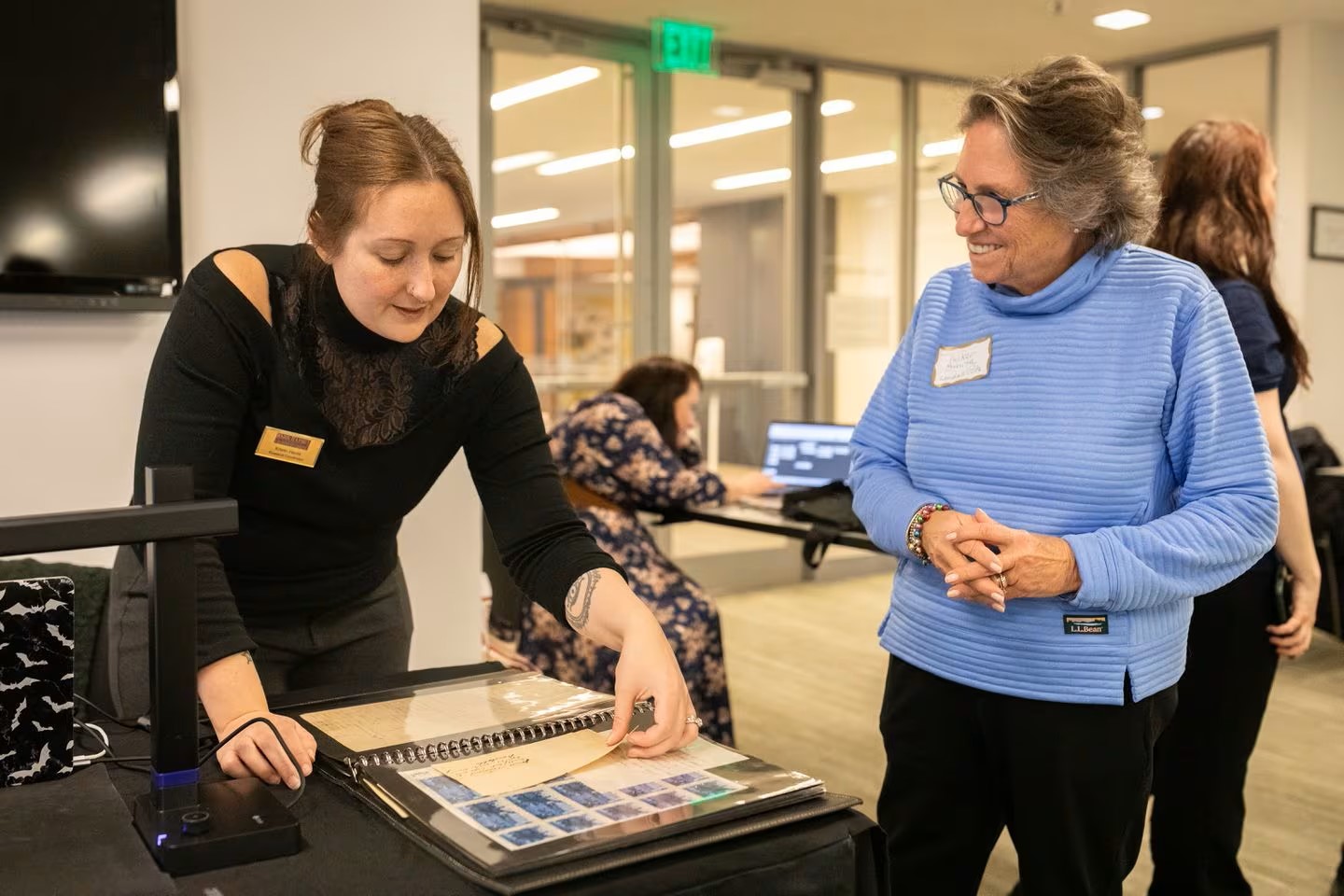The image captures a room inside a building, illuminated by horizontal fluorescent lights on the ceiling. At the forefront, there are two women at a black desk with name tags. The woman on the left, donning gray pants, a long-sleeved black shirt, and a scarf, is examining a binder filled with what appears to be pictures or patterns in blue. She has brown hair and is engrossed in her task. Next to her is an older woman wearing black pants, a slouchy, powder-blue sweater, and a temporary sticker name tag. Her gray and black hair is short, and she is observed standing beside the woman with the binder.

In the background, another lady in a blue and pink floral dress is seated at a different desk, engaged in a phone conversation while working on a computer. Also present is a woman in what appears to be a nurse's outfit, standing further in the room. This room has windows and a grayish hardwood or tan carpeted floor. An exit sign is visible above a set of glass doors, and a TV is mounted on the wall to the left. The black desk appears to have additional items, perhaps a speaker, microphone, or another laptop.